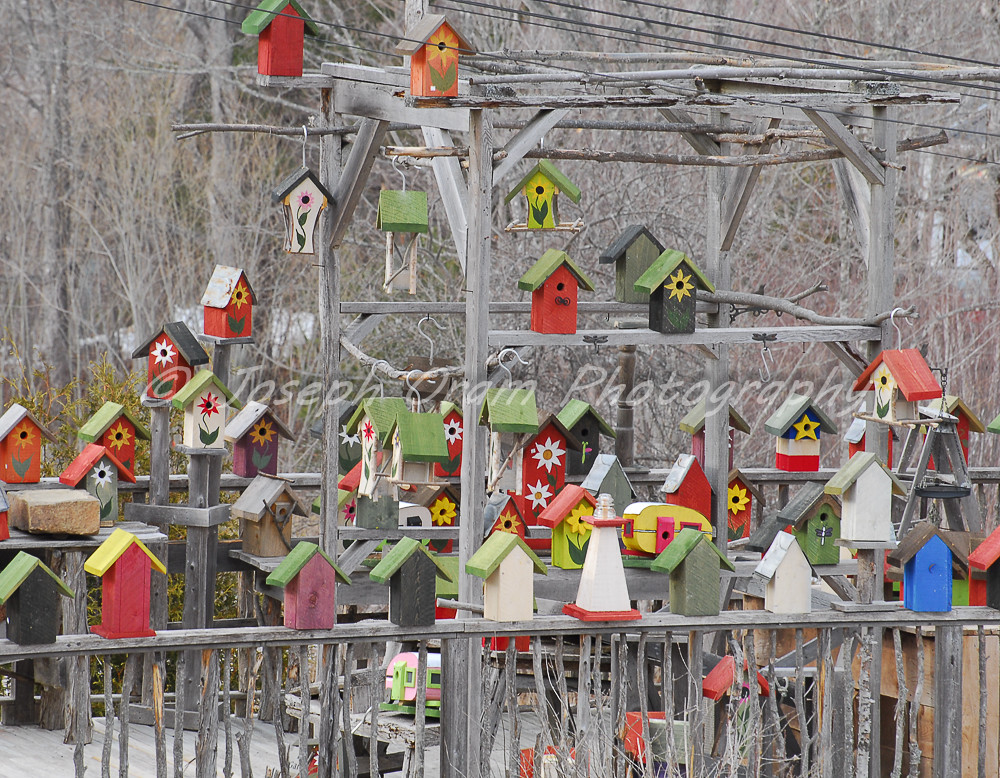This photograph depicts a vibrant display of over two dozen small birdhouses, all meticulously arranged on a rustic, light gray wooden deck with a weathered, faded finish. The birdhouses, varying in hues of red, yellow, white, blue, black, and dark green, share a common design: each is adorned with flowers or sunbursts around their single bird holes. Most birdhouses feature green roofs, while others have roofs in shades of red, yellow, or white. They are mounted on brown pillars, an old fence, and a trellis-like arbor, adding to the charm of the setting. The arbor stands with four legs, supporting additional platforms and branches where more birdhouses hang. Towering, leafless trees form the backdrop, their brown branches poking through the scene. In the center of the image, partially transparent white text reads "Copyright Joseph Oram Photography," marking the image's creator. The outdoor scene is captured during an overcast day, adding a serene, soft light to the quaint birdhouse collection.